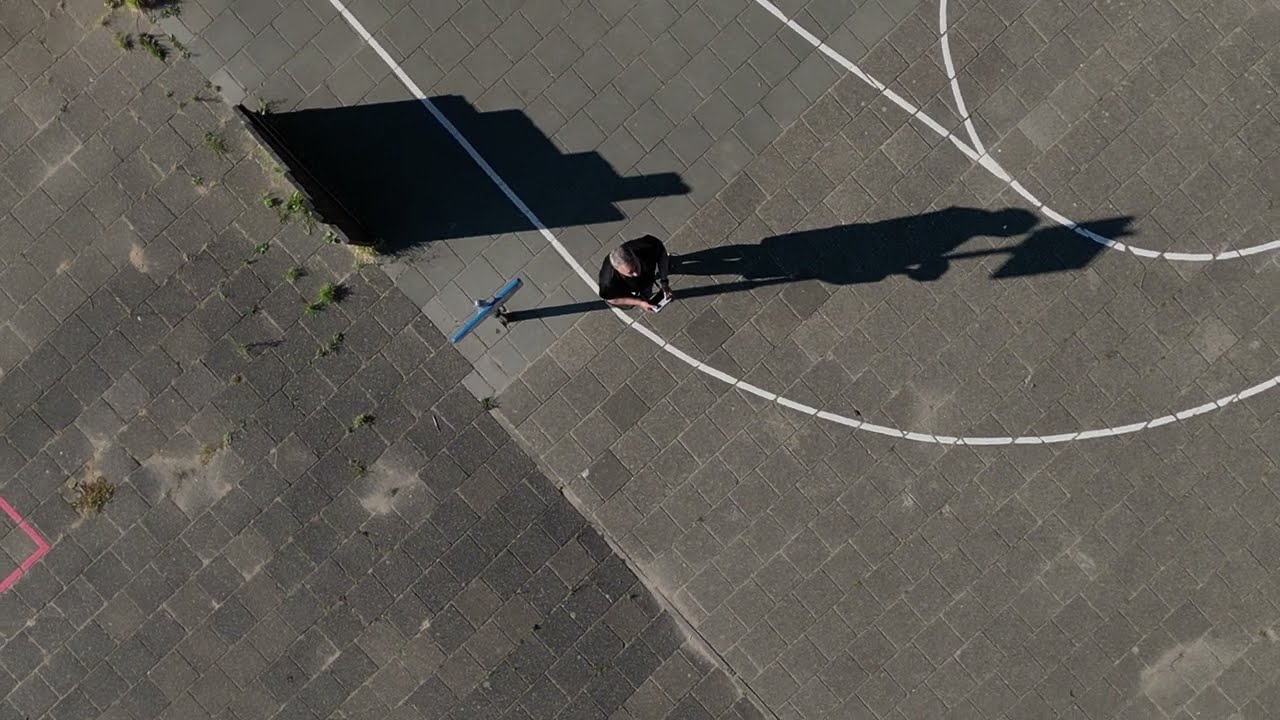This aerial photograph captures a man standing alone on a gray and brown brick pavement, centered in the upper half of the horizontally aligned rectangular image. Viewed from directly above, the scene appears lit by daylight, casting subtle shadows. The man, with short gray hair, is dressed in a black short-sleeved shirt and is holding a device, likely a drone controller or a cell phone. A street sign, blue in color, is attached to a pole just to his left. Distinctive white, curved lines run through the bricks, evoking the outline of a court or specific path markings. A few patches of weeds are visible among the bricks on the left side, adding a touch of greenery to the predominantly gray and brown scene. There are no other people, vehicles, or buildings present, emphasizing the solitary figure and the structured simplicity of the outdoor environment.